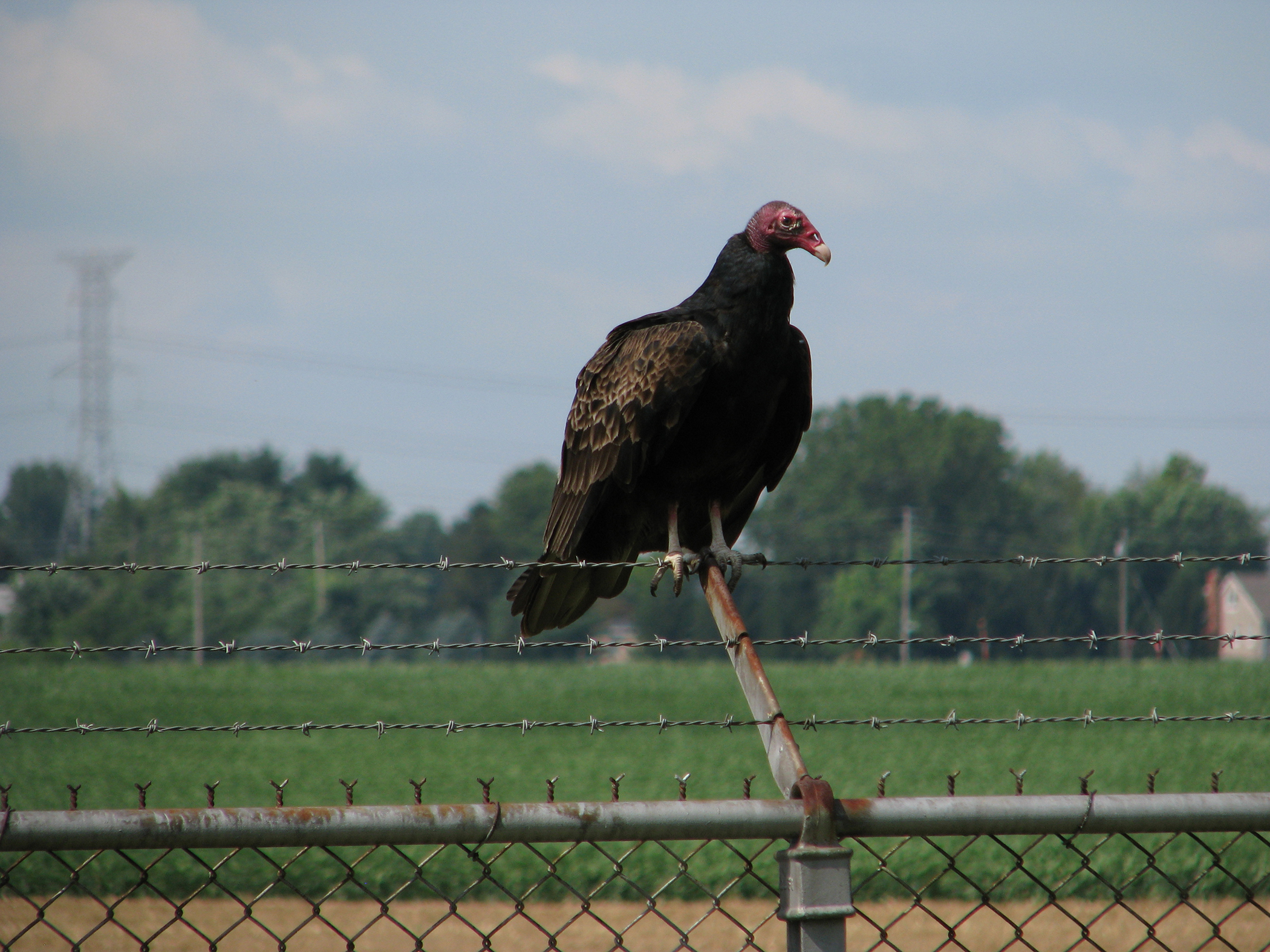In the photograph, a large vulture with a bald, reddish head and a pale beak is perched confidently on an old, rusted barbed wire fence. The bird's predominantly black feathers are interspersed with subtle brown and golden patterns, giving it a rugged and majestic appearance. Its sharp talons clutch the supporting metal piece of the fence, rather than the barbed wire itself, while it gazes directly into the camera. The background features a picturesque scene with vast stretches of green grass, a forest filled with lush trees, and a tranquil blue sky dotted with a few drifting clouds. Among these elements, power lines and an electrical tower subtly blend into the scenery, accompanied by the distant silhouette of a small house with a chimney, enhancing the rustic charm of the setting.